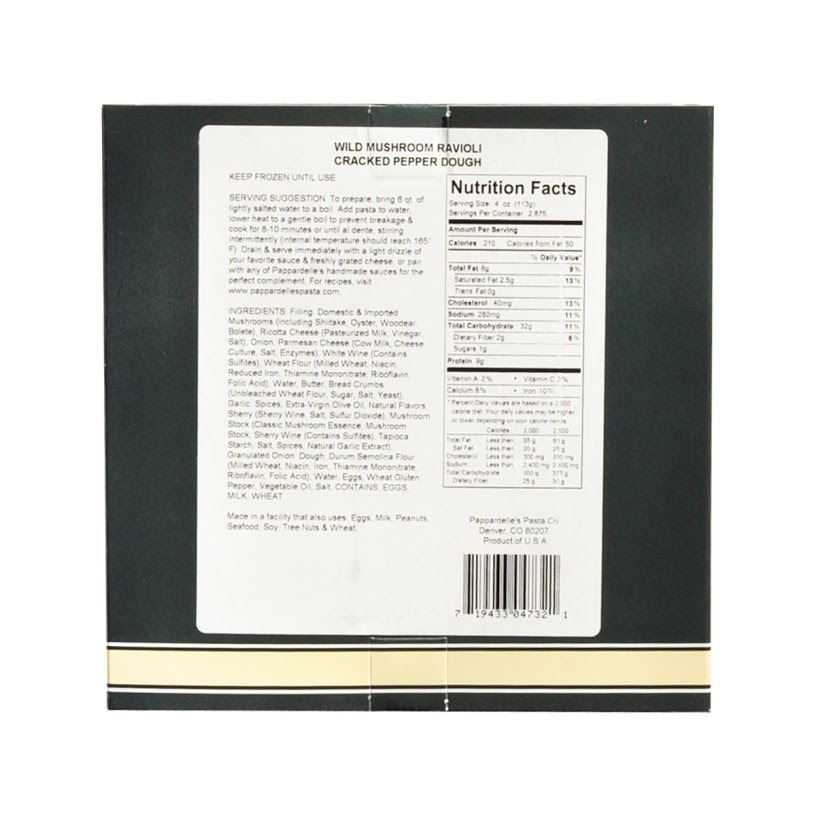The image showcases the back of a food packaging, specifically for "Wild Mushroom Ravioli with Cracked Pepper Dough." The packaging design features a hunter green background with a series of decorative stripes at the bottom, including a thin white stripe, a thin black stripe, a thicker cream-colored yellow stripe, another thin black stripe, and finally a white stripe. The nutrition label, prominently placed in a white rectangular box with rounded edges, displays vital information in black text.

At the top of the label, it reads: "Wild Mushroom Ravioli, Cracked Pepper Dough, Keep Frozen Until Use." Below, the nutrition facts are listed: Serving size is 4 ounces with 2.875 servings per container. Each serving provides 210 calories, 50 of which are from fat. It includes 6g of total fat (9% DV), 2.5g of saturated fat (13% DV), 0g of trans fat, 40mg of cholesterol (13% DV), 280mg of sodium (11% DV), 32g of total carbohydrates (11% DV), 2g of dietary fiber (6% DV), 1g of sugars, and 5g of protein. Vitamins and minerals are listed as Vitamin A 2%, Vitamin C 2%, Calcium 8%, and Iron 10%.

Further down, preparation instructions advise to bring 6 quarts of lightly salted water to a boil, add pasta, lower to a gentle boil, and cook for 8-10 minutes until al dente, ensuring an internal temperature of 165°F. Instructions also suggest serving immediately with a light drizzle of favorite sauce and freshly grated cheese, or pairing it with any handmade sauces. For more recipes, one can visit www.herberdalepasta.com.

At the bottom of the label, it mentions "Pepper Deli's Pasta Company, Denver, Colorado, 80207, Product of USA," and includes a barcode for scanning.